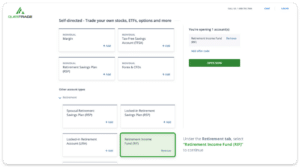Here is a detailed caption for the described image:

---

The image is a screenshot of a website, displayed at a very small resolution making the text unreadable. The website features a clean, white background. In the upper left-hand corner, there is a green icon resembling a mountain. Directly beneath the icon, there are two words: one in green and the other in black. The body of the website is populated with a line of black text spanning across the width of the page. Below this text line, there are four rectangular boxes, each containing some text. Adjacent to these boxes, there is a longer rectangular box with text inside and a dark green box positioned underneath it. 

Then, there is another content section which starts with a black title, followed by four aligned rectangular boxes, all containing black text. Notably, the fourth box on the lower left is filled with green color and outlined in green. On the right side of this section, there is a text in black followed by green text underneath. At the top of the webpage, there are a few words in black, while two words stand out written in blue. Despite the detailed structure, the small size of the image renders the actual text content unreadable.

---